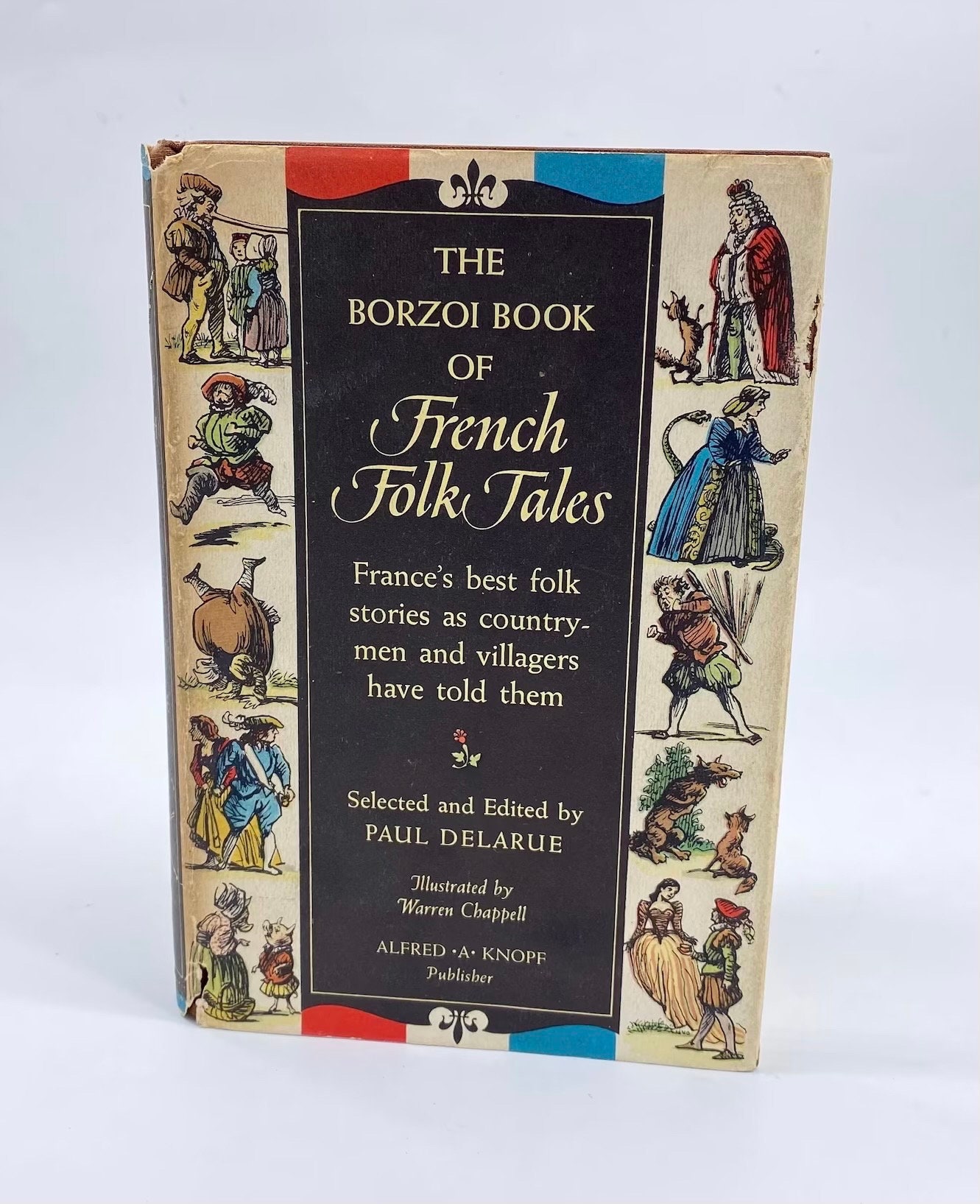This image is a photograph of the front cover of a vintage book titled, "The Borzoi Book of French Folk Tales, France's Best Folk Stories as Countrymen and Villagers Have Told Them." The book appears worn and shows signs of age with some rips and tears along its cover. The central area of the cover features a rectangle of black that prominently displays the title and the book's details: selected and edited by Paul DeLaharie, illustrated by Warren Chappell, published by Alfred A. Knopf.

The black rectangle is flanked by two faded stripes, red on the left and blue on the right. Along both sides of this rectangle are old-fashioned illustrations related to the folk tales within. On the left side, there are images of a man with an extraordinarily long nose talking to children, a man running, and various other characters including a king conversing with a dog. The right side also features detailed illustrations like a woman in blue with a snake near her, a man holding sticks, and characters such as a wolf, a fox, and a couple at the bottom. These colorful and intricate drawings collectively evoke the charm and whimsy of traditional French folklore.